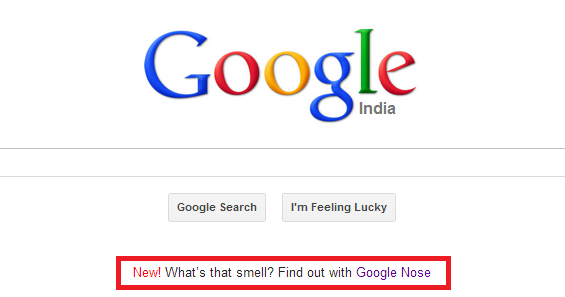This screenshot captures an older version of the Google search engine homepage, evident from the use of outdated fonts indicative of a design from several years prior. In the center, the iconic Google logo is prominently displayed against a clean, white background. The logo itself retains its classic color scheme: a blue "G," red "O," yellow "O," lowercase blue "g," green "l," and red "e." This particular version is localized for India, as indicated by the word "India" in gray font beneath the "l" and "e."

The search box spans the width of the page, delineated by two very thin gray lines. Below this box are two light gray rectangle buttons. The button on the left is labeled "Google Search" and the one on the right reads "I'm Feeling Lucky." Further down, a distinctive highlight is evident: a red-drawn rectangle encasing text that reads "New!" in bold red font, followed by "What's that smell?" in gray font. It continues with "Find out what Google knows," alluding to an April Fool's joke that was part of Google's playful tradition for that year.